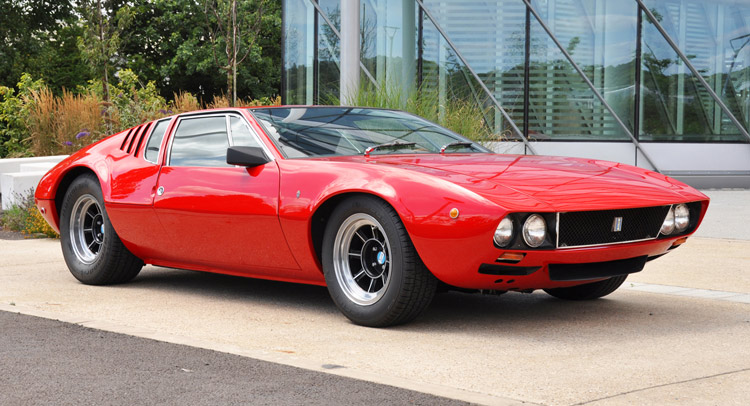This image showcases a classic, bright red sports car, likely an Italian model from the 1960s or 1970s. The car, which features a distinctive long hood, muscular front with four headlights, and a black grille, is parked on a beige-colored ground. Its chassis sits very low to the ground, highlighting its sports car design. The vehicle, which appears to be a two-door model with a wide windshield, is oriented with its front facing right. No one is inside the car. In the background, there is a modern building characterized by numerous large, clear glass windows. Flanking the building to the left, a cluster of green trees is visible, adding a touch of nature to the urban setting. The scene suggests the car might be displayed near a classic car dealership or a similar establishment.